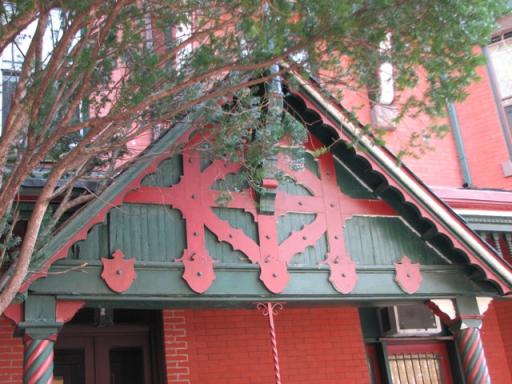In the image, we see a rustic street storefront or barn, characterized by its unique color scheme and decorative elements. The building, primarily composed of dark pink painted bricks, features a prominent entryway with a porch and a peaked roof. The peaked roof is adorned in a dark hunter green color with pink trim, visually tying into the overall building's color palette. 

Two striking pillars frame the entryway, each spiraling diagonally with green and pink stripes. Above the porch, there is a triangular frame, predominantly green, adorned with a red emblem that hints at designs reminiscent of a bridge or even a nod to Superman's badge. 

In the upper left corner of the image, a tree extends its branches and foliage, adding a touch of nature to the scene. The building appears to have multiple doors and windows, indicating it could be a business or a residential house. Behind the main structure, another building with a similarly colored roof is visible, adding depth to the picturesque setting.